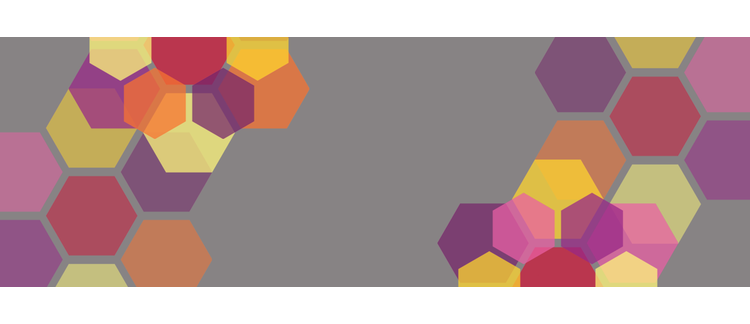The image depicts an abstract, geometrically styled art piece with a dark gray background. The central feature is a long, narrow, purplish-gray rectangle. Surrounding this rectangle are several slightly translucent hexagons in an assortment of colors, including purple, red, yellow, orange, and pink. These hexagons are arranged into two vertical columns on the left and right sides of the rectangle, leaving the center predominantly gray. 

In the top right corner, a sequence of hexagons displays partial images of a dark pink, yellow, and dark purple hexagon, alongside the full image of a red hexagon. On the bottom left corner, there's a partially visible purple hexagon. The style of the hexagons is simplistic and uniform, resembling clipart, and they are about one inch wide. Some hexagons overlap slightly, creating a layered effect, while others are more evenly spaced, especially towards the edges, where the gray background remains visible between them. This creates a honeycomb-like pattern, emphasizing the abstract and minimalistic composition of the piece.